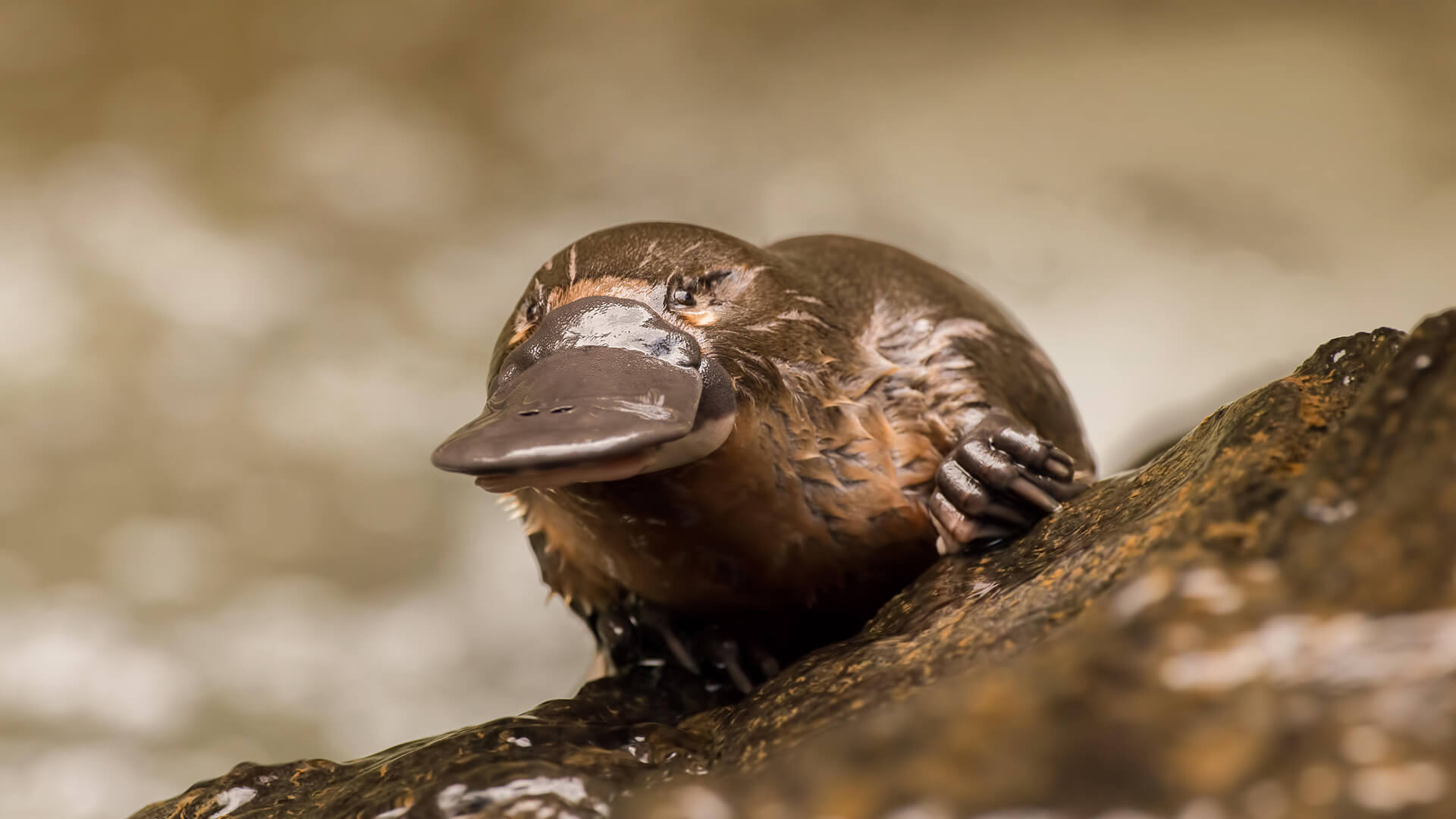This photograph features a close-up view of a baby platypus centrally positioned on a wet, brown rock that inclines from the bottom left to the middle right of the image. The platypus is notable for its elongated body, light brown mixed with an orange underbelly, and a distinctive grayish-brown bill. It is looking towards the camera with its small, visible eyes. Its tiny, pointy claws cling to the rock, which glistens in the sunlight. The animal appears shiny and wet, as if it has just emerged from the water. The background is completely out of focus, consisting of blurred white, tan, brown, and gray hues, creating a sense of depth that emphasizes the platypus and the rock. There is no text associated with the image.